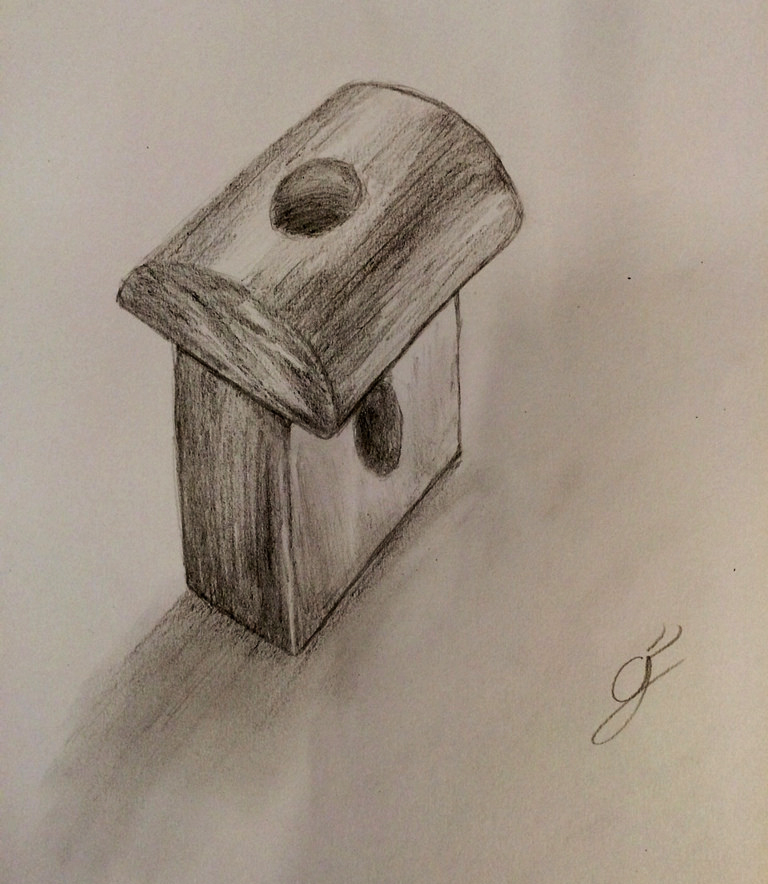The artwork depicted in this image is a monochromatic piece created using either black colored pencil or graphite. The artist has employed extensive shading techniques to add depth and dimension to the drawing, which is rendered on plain white, unlined paper. In the bottom right corner, the artist has signed the work with a unique symbol that combines a cursive "G" and a lowercase "f."

The drawing showcases an intricately shaded wooden sculpture. The base of the sculpture is a wooden square, heavily shaded on the left side to create a sense of depth and dimensionality, with a darkly shaded hole positioned centrally within it. On top of this square base rests another wooden piece, this one rounded at the top. It also features a carved hole in its middle, highlighted by the detailed shading that gives the entire piece a realistic and textured appearance. The careful attention to shading highlights the craftsmanship and detail of what appears to be a carved wooden structure.